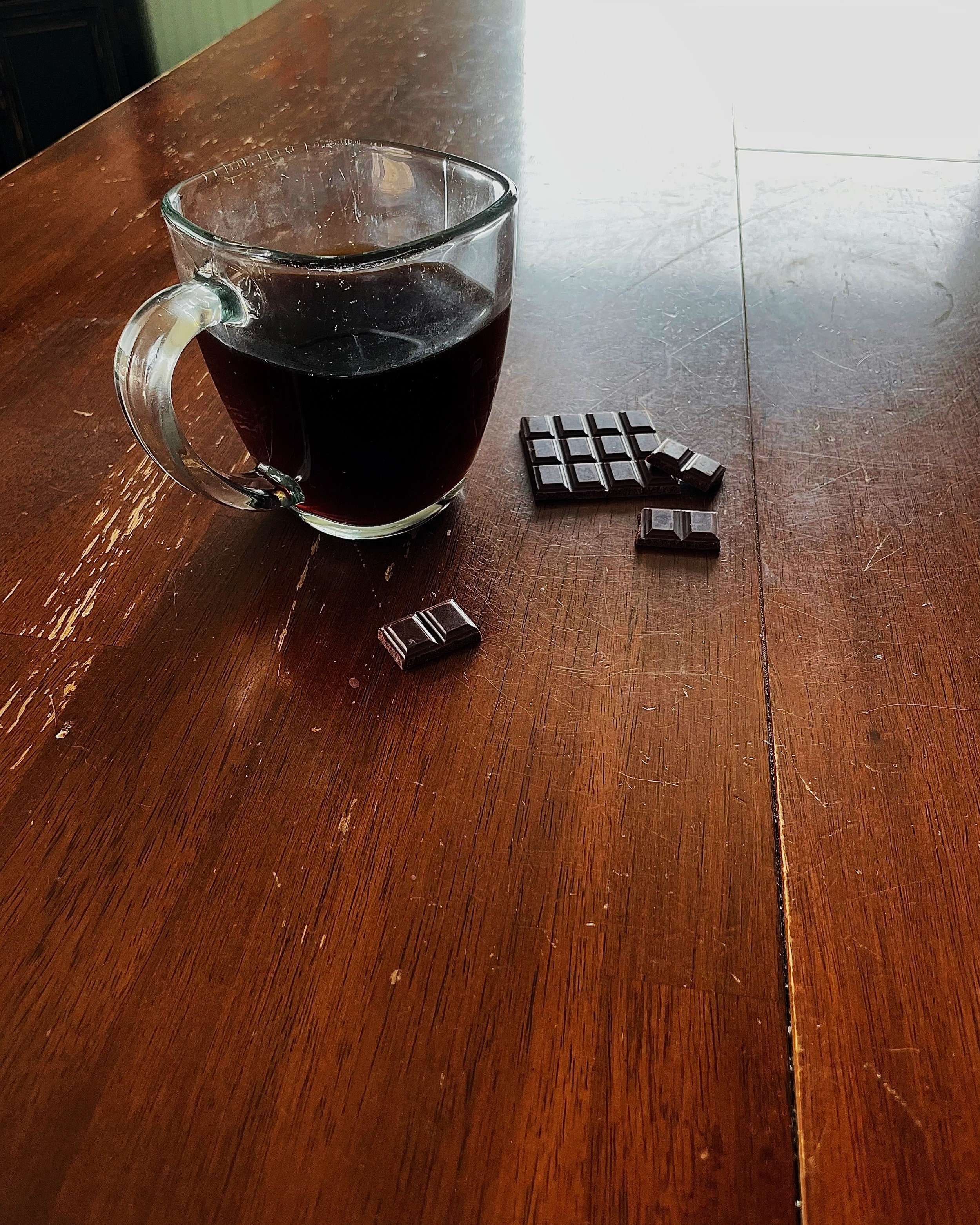In this color photograph, a clear glass mug with a handle sits on a worn, medium-brown wooden table, characterized by visible rings and patches where the varnish has peeled off. The mug is partially filled with a dark brown liquid, likely black coffee. Next to the mug, there's a chocolate bar that's broken into pieces. A large segment remains intact, while the smaller adjacent chunks hint at the original division of the bar, suggesting it may be a Kit-Kat or similar chocolate. On the far left of the image, the table ends near a lime green wall. The scene is devoid of people, emphasizing the solitary nature of someone enjoying coffee with chocolate. The image, taller than it is wide, captures a sense of everyday simplicity.